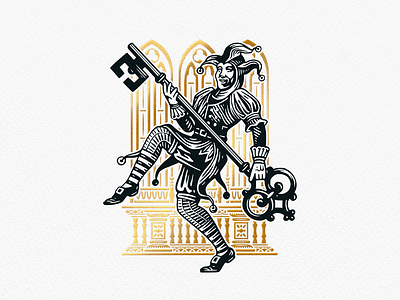The image is a detailed illustration of a court jester or joker, akin to the ones depicted on playing cards. The jester, dressed in a traditional outfit complete with a headpiece featuring three prongs ending in bells, is the central focus. He wears a skirted dress adorned with bells, striped socks, and black shoes with buckles, and his hands are gloved. The jester holds an oversized, ornate key with both hands – a key nearly as large as he is. His posture suggests he is in mid-dance, one leg kicking upward, leaning back, and with a slightly serious facial expression. Adding to the enchantment, the jester is placed against a white backdrop with a golden, ornate design that resembles church windows, evoking a sense of luxury and elegance around him. The image is rendered in black and white, except for the golden background detailing.